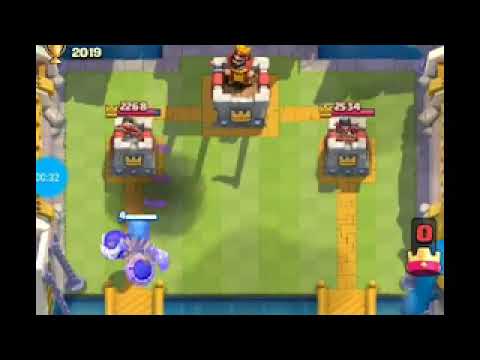The image is a simple, 2D composition primarily featuring three main sections arranged vertically. At the very bottom, there is a black rectangle occupying about one-eighth of the image's height. Directly above this bottom section is a goldish-yellow stripe that spans approximately one-third of the image. This stripe has a gradient, starting lighter at the bottom and darkening as it ascends. The top portion, making up roughly two-thirds of the image, is another black rectangle, the same color as the bottom section. The overall structure resembles a flag-like pattern with a large black area on top, a goldish-yellow band offset towards the lower part of the image, and a smaller black strip at the bottom. The image is devoid of text, figures, or any other elements, and consists solely of the colors black and yellow.